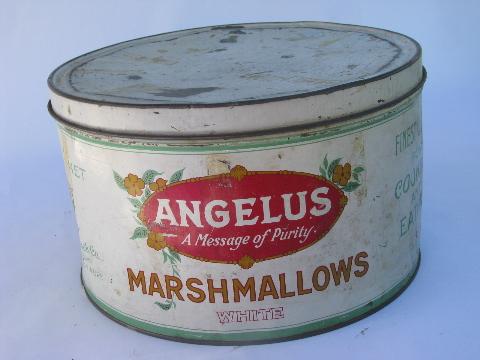This image depicts an old, squat, and round tin can used to store marshmallows, originating from the early 1900s. The can features a white background, although it appears aged, with evident rust spots, dirt, and some scuffs, particularly noticeable on the top lid. A red lozenge-shaped logo prominently displays the word "ANGELUS" in white capital letters, accompanied by the phrase "a message of purity." Surrounding the logo are orange flowers and greenery, along with other decorative elements in an Art Nouveau style. Below the logo, the word "marshmallows" appears in gold leaf lettering with red accents, followed by the word "White." The can also includes some partial, hard-to-read text in a stylish font, likely saying something like "finest gourmet something." A small dent is visible, adding to the vintage charm of the tin. The can is positioned against a white background in the image.